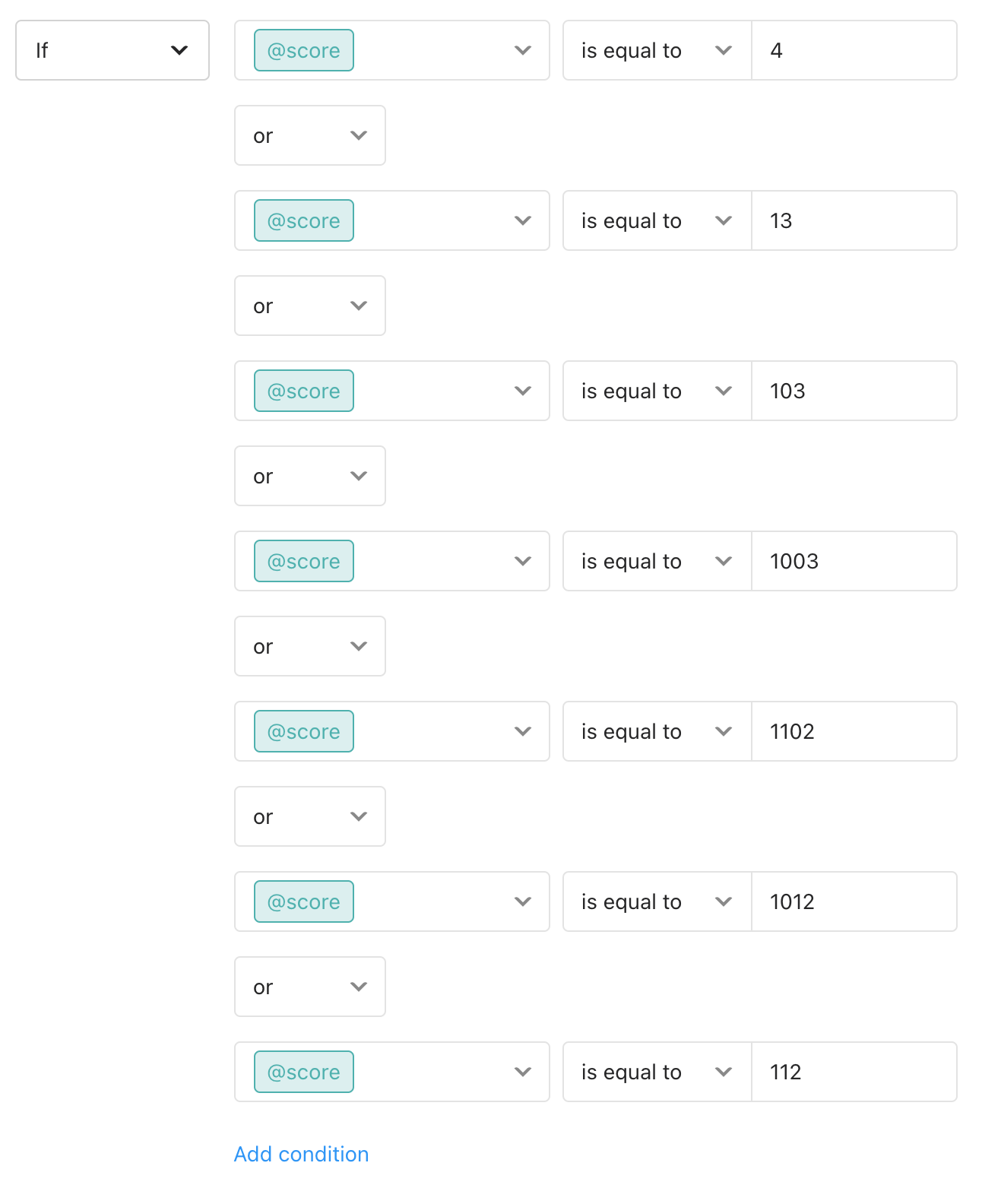On this page, there is a white background. On the left side, there is a small box outlined in gray with the text "IF" and a down arrow. On the right, there is a white box containing several elements arranged vertically:

1. A blue highlighted "score" next to a down arrow, with text indicating "is equal to".
2. A series of conditions, each separated by "OR":
   - First condition: "score" (highlighted in blue) "is equal to" a drop-down menu, with the value '13'.
   - Second condition: "score" (highlighted in blue) "is equal to" a drop-down menu, with the value '103'.
   - Third condition: "score" (highlighted in blue) "is equal to" a drop-down menu, with the value '1003'.
   - Fourth condition: "score" (highlighted in blue) "is equal to" a drop-down menu, with the value '1102'.
   - Fifth condition: "score" (highlighted in blue) "is equal to" a drop-down menu, with the value '1012'.
   - Sixth condition: "score" (highlighted in blue) "is equal to" a drop-down menu, with the value '112'.

At the bottom of the box, there is an option labeled "add condition" highlighted in blue.

This layout appears to be part of a form or a query builder interface designed for setting conditions based on specific score values.